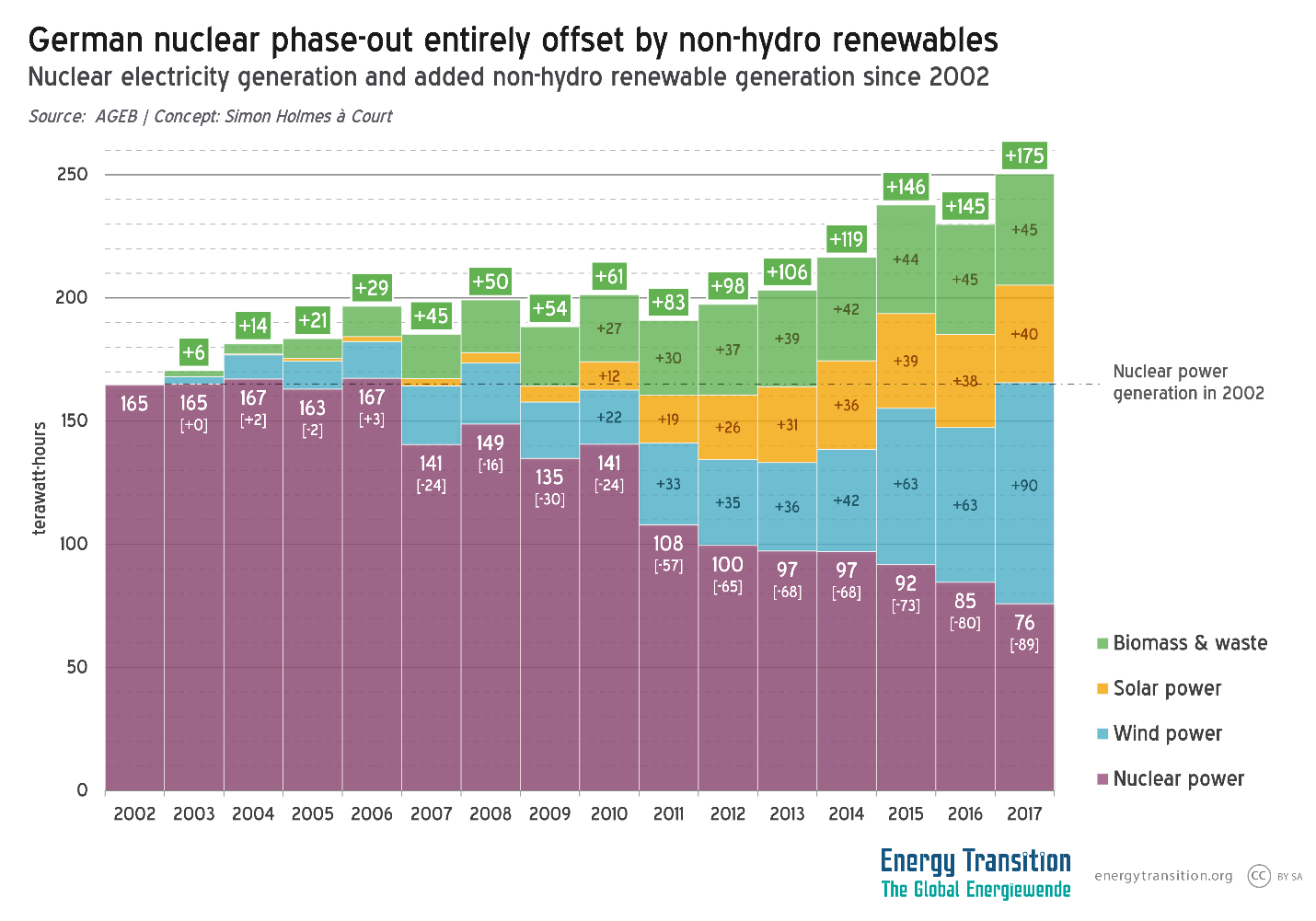**Detailed Caption:**

The image is a bar chart illustrating energy generation trends in Germany over time, particularly focusing on the impact of the phase-out of nuclear power and the rise of non-hydro renewable energy sources. The chart is rectangular, with its width greater than its height, and features a solid white background. At the top, the title is displayed in multiple lines of black printed text. The top line reads: "German Nuclear Phase-Out Entirely Offset by Non-Hydro Renewables." The second line states: "Nuclear Electricity Generation and Added Non-Hydro Renewable Generation Since 2002." Below this, the third line provides the source: "Source: AGEB / Concept: Simon Holmes à Court."

Dominating the image is the detailed bar chart, using four colors to represent different energy sources: green, yellow, blue, and purple. According to the color legend in the bottom right corner, green indicates biomass and waste, yellow represents solar power, blue signifies wind power, and purple denotes nuclear power. Each color highlights the evolving contributions of these energy sources over the years.

In the bottom right corner of the image, there is text that reads: "Energy Transition: The Global Energy Wende."